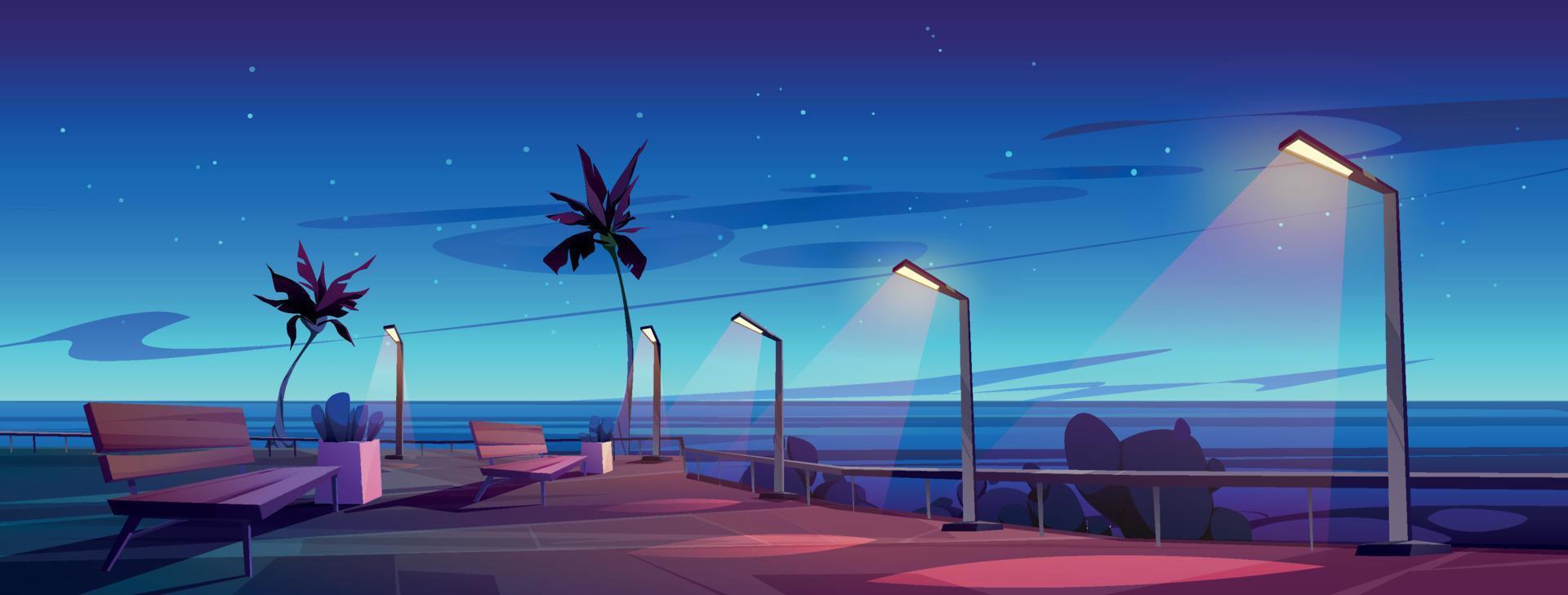This is a computer-generated image depicting a wide, expansive boardwalk or deck overlooking the ocean at night. The scene is bathed in various shades of blue with a transition from dark to light blue in the sky, which is dotted with white and light blue stars. The sky also features a few scattered dark blue clouds, adding to the night-time ambiance. The deck, characterized by its reddish-brown wood and dark brown concrete sections, is lined with a small gray railing.

On the left side of the foreground, there are wooden benches, one prominently in the front and another slightly further back. Between these benches stands a white, rectangular planter box with a small plant. The deck also features purple and black palm trees, adding a tropical feel to the scene. Tall, silver street lights line the right edge of the boardwalk, casting a golden light downwards and creating a soft, warm glow against the cooler tones of the deck.

Beyond the railing, the deep blue expanse of the ocean stretches out, meeting the sky in the background. On the right side, beyond the railing, some rocks are visible, adding to the natural coastal elements of the image. Overall, the comprehensive details and color variations contribute to a serene, picturesque night-time beach scene.